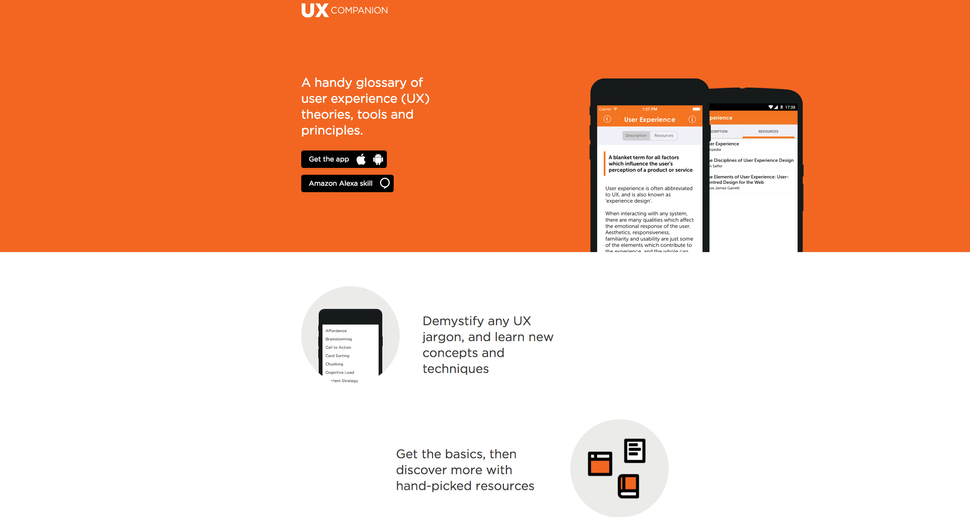This image appears to be a digital poster or informational sign promoting a user experience (UX) resource application. At the top, an orange banner prominently displays the title "UX Companion" in white text, slightly left of center. Beneath the title, the tagline "A handy glossary of user experience (UX) theories, tools, and principles" is written in white.

Below this, two black bars offer further actions. The first bar, with the text "Get the App" in white, presents icons for Apple and Android, suggesting the app is available on both platforms. The second bar reads "Amazon Alexa Skill" in white text, accompanied by a white speech bubble icon on the right, indicating compatibility with Amazon's voice-activated assistant.

To the right of the text, there are two cell phone visuals, showcasing the app's interface and user experience on mobile devices. This visual aid helps to provide a preview of the app in use.

The larger white section below these visuals features informative text and graphics. On the left, a gray circle contains a black outline of a cell phone with a list of words that are too small and blurry to identify, accompanied by the phrase "Demystify any UX jargon and learn new concepts and techniques."

Toward the bottom right of this section, another gray circle depicts an icon of three web pages stacked together. The text next to it reads, "Get the basics, then discover more with hand-picked resources," emphasizing the comprehensive nature of the UX resources provided.

The overall design effectively communicates the purpose and functionality of the UX Companion app, making it clear that it is a valuable tool for learning and mastering UX principles.